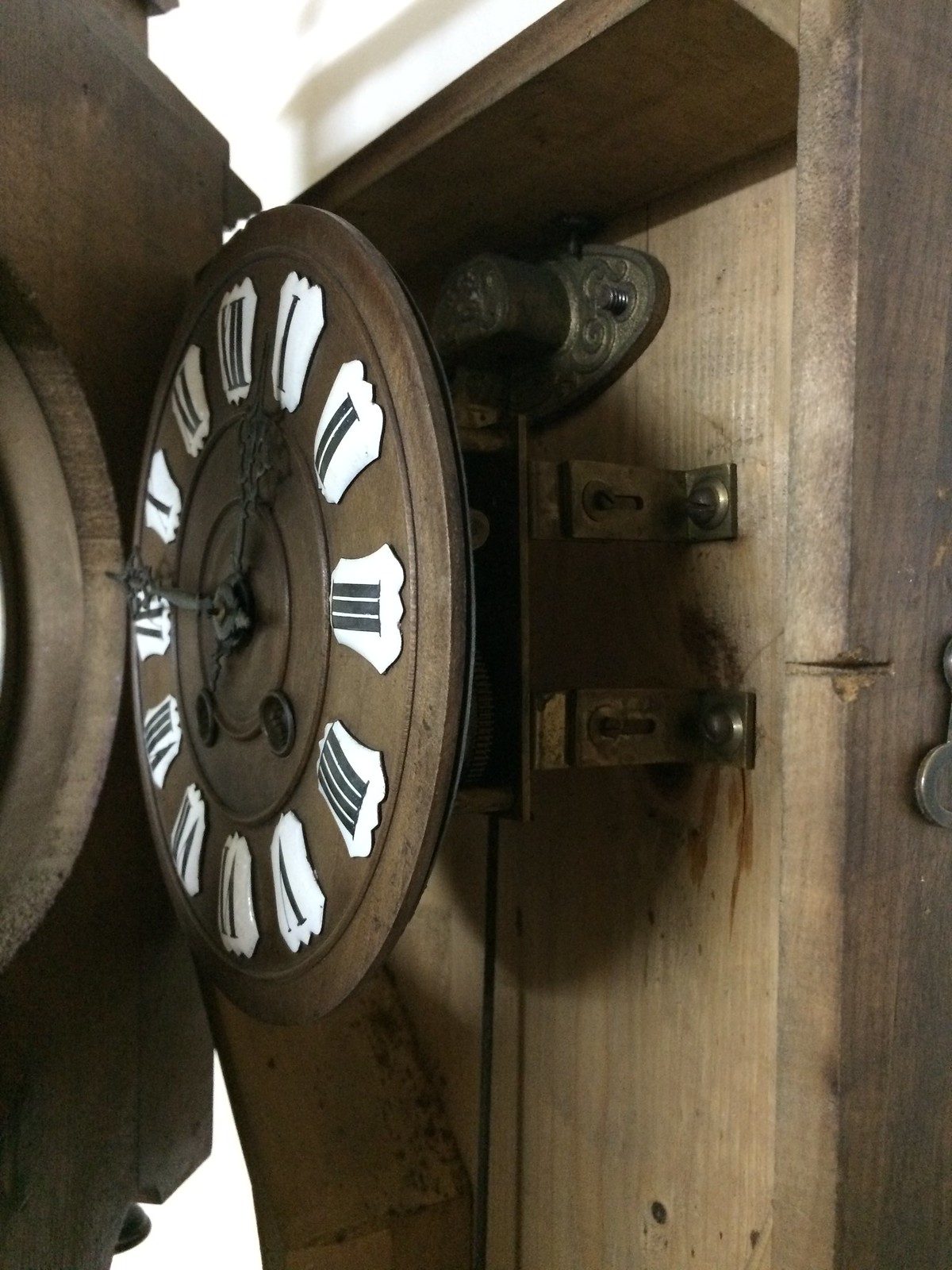A detailed close-up image depicts an ornate clock encased within a polished brown wooden box, which is affixed to a pristine white wall. The clock's face is elegantly elevated a few inches from the backdrop of the box, creating an intricate, dimensional effect. Surrounding the clock face, there are meticulously arranged white markers, each bearing black Roman numerals to denote the hours. Complementing these features, the clock's hands are crafted in a rich brown hue, blending seamlessly with the wooden aesthetics. To the left of the clock, there's a notable wooden door that appears designed to enclose the timepiece. This door aligns perfectly with the clock's circular shape, echoing the same precise dimensions and adding a harmonious symmetry to the overall design.